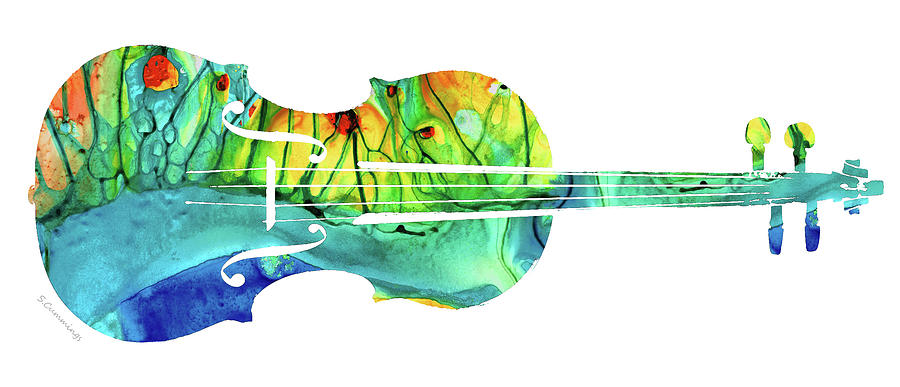This detailed, whimsical drawing depicts a violin or possibly a cello laying on its side, with its neck pointing to the right. The instrument's body features an array of flowing, abstract colors. The bottom section is a dark blue, transitioning to a lighter teal above that. Further up, there is a vibrant mix of teal, orange, and green hues, each section artistically separated by bold black lines. The instrument's strings are depicted as white lines, contributing to its surreal appearance. On the neck, which joins the body with white lines, the top features two points with round, yellow knobs, while the lower part has protruding light blue and dark blue points. The artistic rendering is completed with an indistinct gray signature, prominently featuring the letter "S," located in the bottom left corner. The entire scene is set against a pure white background, adding to the overall contrast and highlighting the vivid color palette of the instrument.